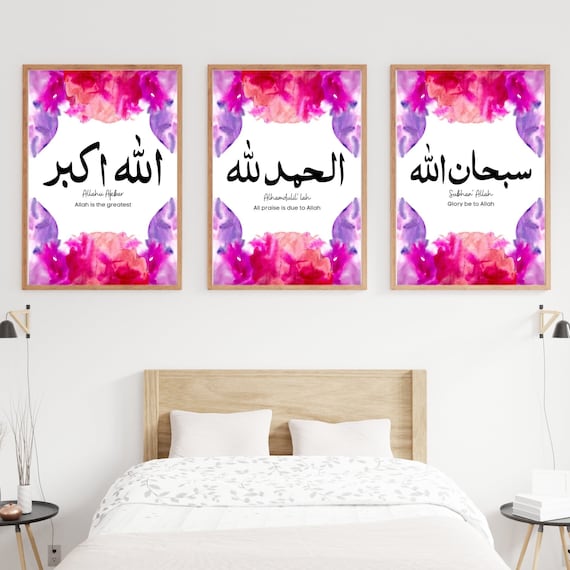This image showcases a contemporary, minimalistic bedroom scene. The focal point is a narrow single bed with a semi-rustic wooden headboard, adorned with two white pillows and a white comforter that features a subtle floral pattern. Flanking the bed are two simple nightstands—small round tables with four wooden legs. Above these nightstands are minimalistic lights, characterized by tiny lamps with black shades and wooden accents, each accompanied by visible black wires. 

Atop the bed's headboard, a white vase with barren branches adds a touch of natural decoration. Dominating the white, beige-toned wall above the bed are three framed prints arranged in a series. Each frame contains a design with pink, purple, and peach floral patterns arcing from the top and bottom. The central part of these prints features bold, black text in an unfamiliar language, possibly Arabic or Farsi, set against a white background. Despite the different texts, the floral border designs in each print are identical, featuring abstract splotches of color that unify the trio. This meticulously staged scene likely aims to highlight the wall prints as the room's central product.